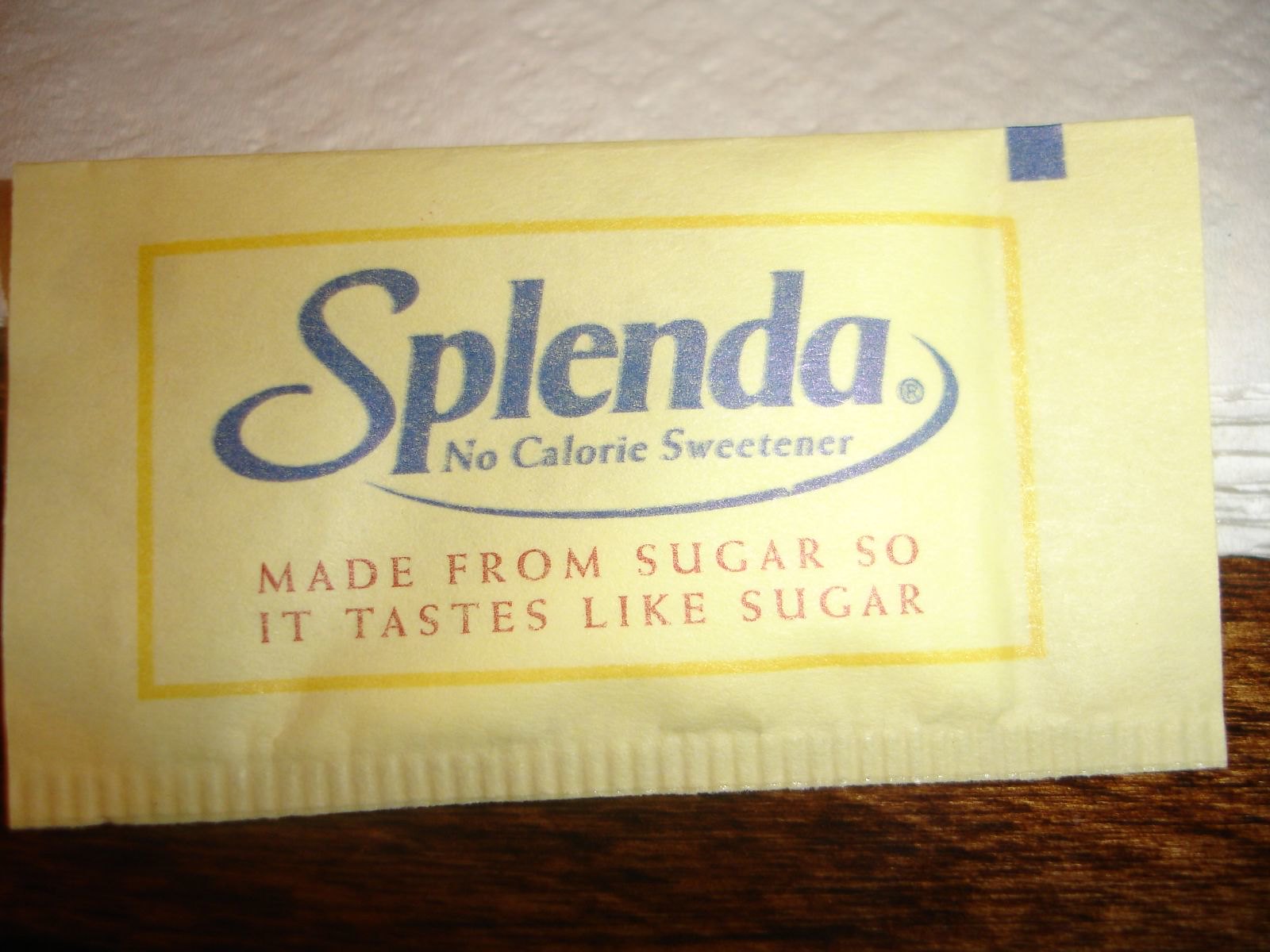The image is a nearly square, close-up, bird's-eye-view photograph of a Splenda no-calorie sweetener packet, typically found in cafes or restaurants. The packet is an off-white, almost light yellow color, and features a prominent blue font with the word "Splenda," followed by "no-calorie sweetener" beneath it. A thin yellow rectangular border surrounds the text. Below this, in smaller red block letters, the packet states, "Made from sugar, so it tastes like sugar." In the upper right corner, a small blue square indicates where to tear the packet open. The packet rests on a dark brown wooden table, where the wood grain runs horizontally, and the top part of the background includes a white piece of kitchen roll or napkin, suggesting the setting is in a coffee shop or restaurant. The lower right corner of the packet also features a copyright symbol.